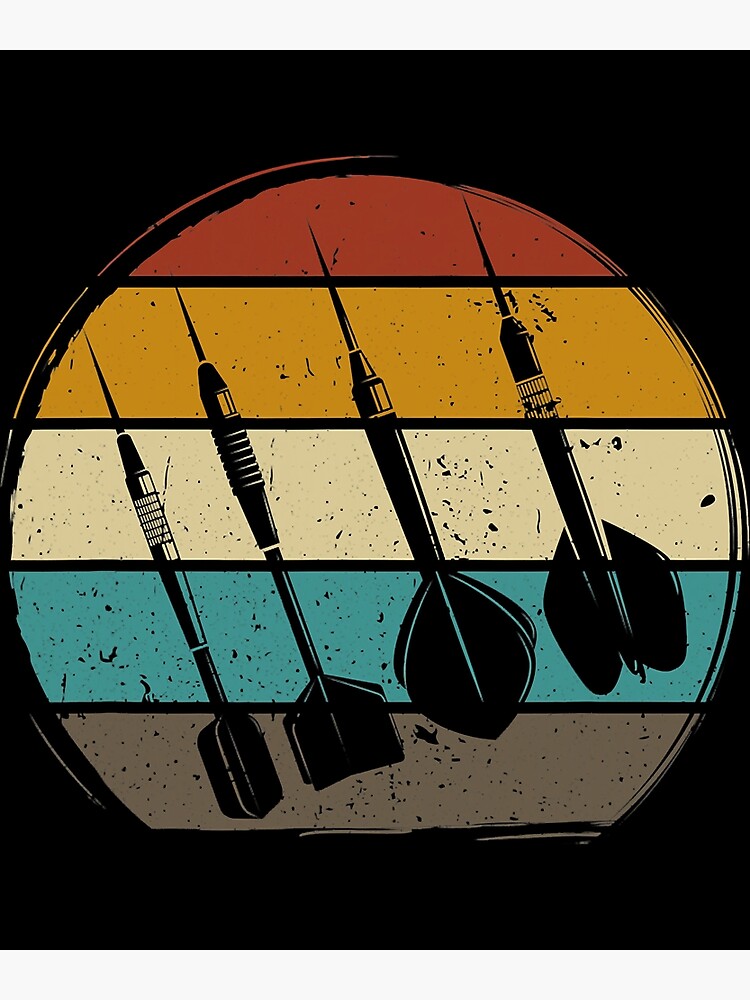The image is an artistic rendering of four distinct darts set against a high-contrast, black background. A multicolored circular feature dominates the forefront, horizontally segmented into stripes of burnt red, burnt orange, white, muted blue, and gray shades. These stripes are speckled with a texture reminiscent of film grain, adding a gritty detail to the design. 

The four darts are oriented with their tips pointing upward, angled approximately 30 to 45 degrees to the left. Each dart varies in design: the leftmost dart is thin with a textured grip and standard dart tail. To its right, the second dart features a four-flagged tail and a slightly larger body with a textured grip. The third dart resembles a quill pen, sporting flared, semicircular tips. The final dart, medium in size, has a textured grip and two discernable tails. The high-contrast elements and diverse dart designs contribute to the dynamic and detailed graphic composition, making it an intriguing visual study of form and texture.